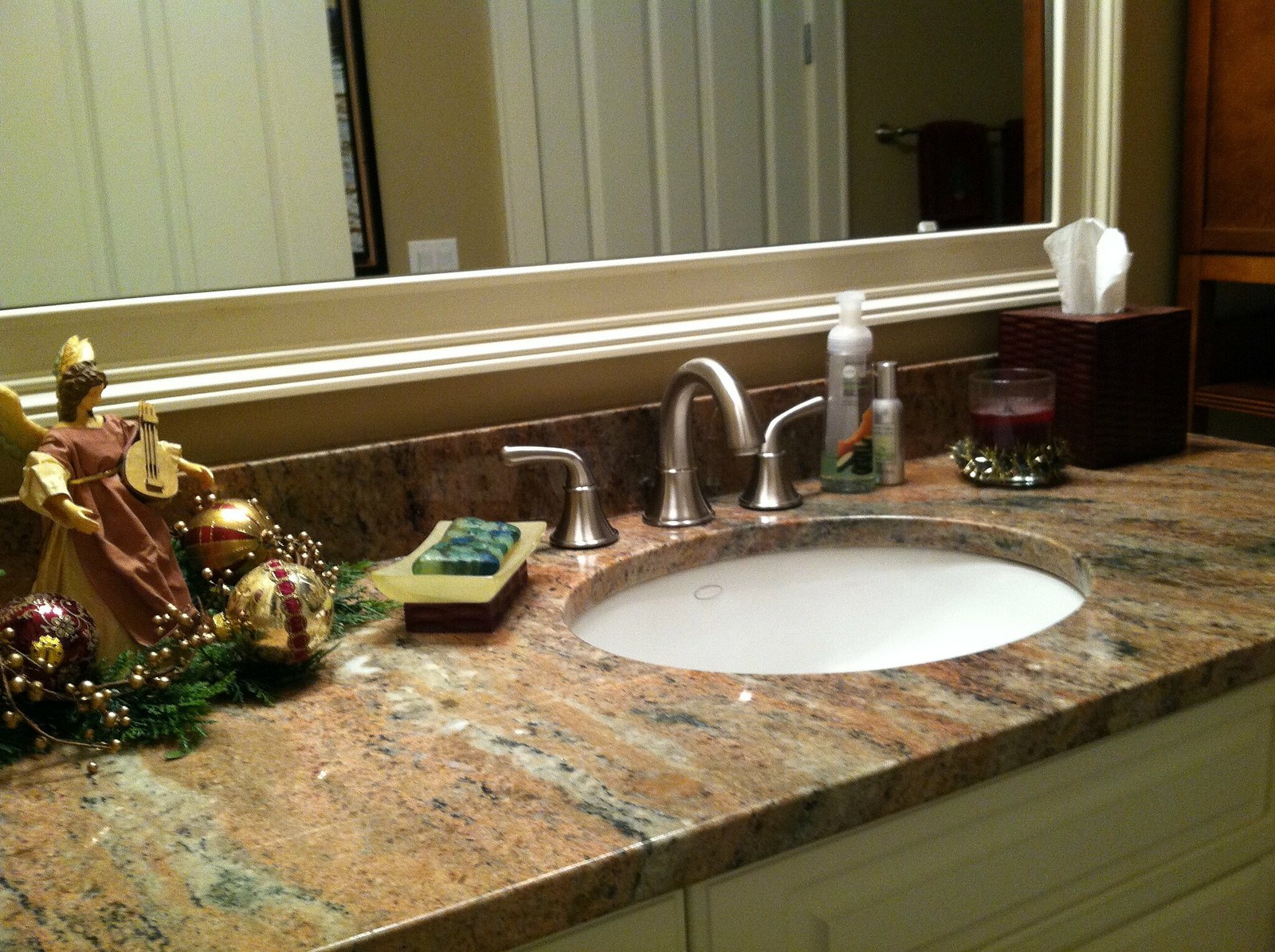This image captures a cozy bathroom scene, likely set during Christmastime. The centerpiece is an oval sink with a marbled countertop in a warm brown-orange hue, interwoven with lighter off-white veins. To the left of the sink stands a delicate angel figurine, adorned with a crown and holding a guitar, surrounded by festive ornaments. This decorative touch complements the specialty soap nearby, presented in shades of green and off-white. The sink is outfitted with sleek, metallic silver fixtures, adding a modern contrast to the rustic countertop.

Also on the countertop is a lit candle in a rich maroon hue, casting a soft glow over the surroundings. A maroon or brown Kleenex box with a protruding white tissue matches the candle’s color scheme. The bathroom walls, visible in the mirror above the sink, are painted a soothing beige, enhancing the room's warm ambiance. To the right, reflected in the mirror, is a towel rack, adding to the room's functional decor. The cabinetry beneath the countertop is finished in an elegant off-white, completing this inviting and festive bathroom setting.